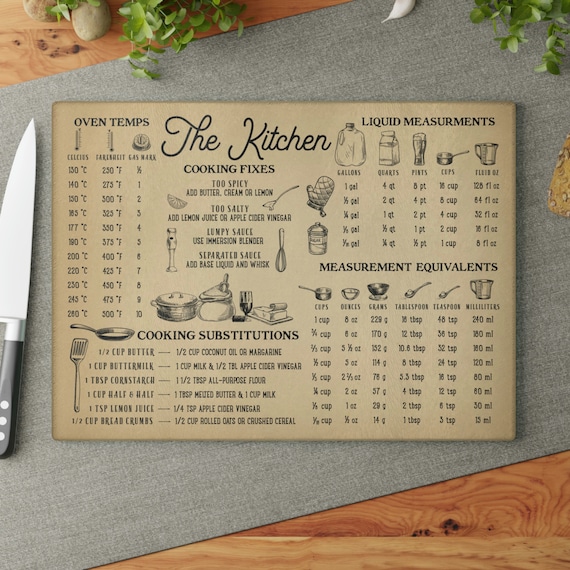The image is a light brown, vintage-style rectangular sign, designed for Instagram or social media, likely as a product photo aimed at kitchen enthusiasts. The sign is placed at a diagonal angle on a medium brown wooden table with a gray table runner beneath it. The sign is adorned with black text and small illustrative icons like a whisk, immersion blender, and oven mitt.

At the top, the sign reads "The Kitchen," followed by "Cooking Fixes," which includes quick tips for common cooking issues: "Too spicy, add butter, cream, or lemon; too salty, add lemon juice or apple cider vinegar; lumpy sauce, use immersion blender; separated sauce, add base liquid and whisk."

The upper left section is labeled "Oven Temps," featuring a conversion chart for Celsius and Fahrenheit temperatures and gas marks for oven settings. Just below this, the "Cooking Substitutions" section offers alternative ingredients, such as using a half cup of coconut oil or margarine for butter, or crusted cereal for breadcrumbs.

The upper right section displays "Liquid Measurements" with conversions for gallons, quarts, pints, and cups. Beneath, the "Measurement Equivalents" section lists various conversions, like one gallon equaling four quarts, eight pints, or sixteen cups. Additional metrics include cups, ounces, grams, tablespoons, teaspoons, and milliliters.

A black-handled butcher knife with a shiny silver blade lies to the left of the sign, and there are leaves on the table's upper left and right corners, adding a touch of rustic elegance to the scene.